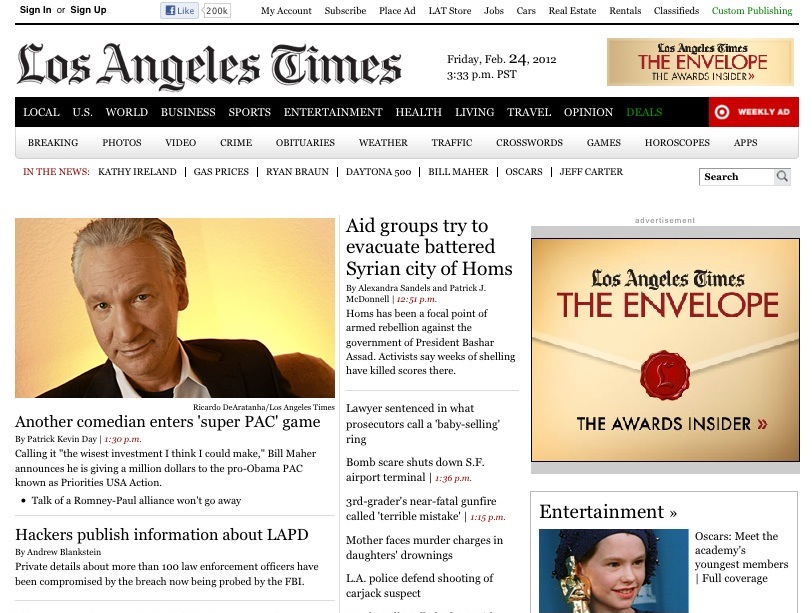This detailed screenshot from the Los Angeles Times online, captured on Friday, February 24, 2012, at 3:33 PM PST, showcases the website's comprehensive layout as viewed on a PC. At the top, user options are available, including sign-up/sign-in, social media engagement, account management, subscription links, and various services like placing ads, LAT store, job listings, car sales, real estate, rentals, classifieds, and custom publishing. The iconic Los Angeles Times logo, styled in Old English text, dominates the header, positioned above the current date and time, displayed in bold on a white background.

Directly below the logo, a call-out for the "Awards Insider" area is highlighted with an envelope icon. The main navigation bar, with a black background, presents a hierarchical menu structure, offering categories such as Local, US, World, Business, Sports, Entertainment, Health, Living, Travel, Options, Deals, and Weekly Ads. Beneath this, a secondary menu lists Breaking News, Photos, Video, Crime, Obituaries, Weather, Traffic, Crosswords, Games, Horoscopes, and Apps.

Under the "In the News" section, trending topics are listed, including Kathy Ireland, Gas Prices, Ryan Braun, Daytona 500, Bill Maher, the Oscars, Jeff Carter, and a search field for user queries. 

The screenshot features three content columns, with the leftmost column showcasing an image of Bill Maher under the headline, "Another comedian enters Super PAC game." Further down, a second story reads "Hackers publish information about LAPD." The center column highlights international news with a report on aid groups attempting to evacuate battered Syrian homes in Homs.

On the right, the "Awards Insider" area recurs, marked by the envelope icon and the section name "The Envelope," branded with a faux wax seal stamped with an "L." Below this, an entertainment piece features a young child under the headline "Oscars: Meet the academy's youngest members," pointing to full coverage of the Oscars.